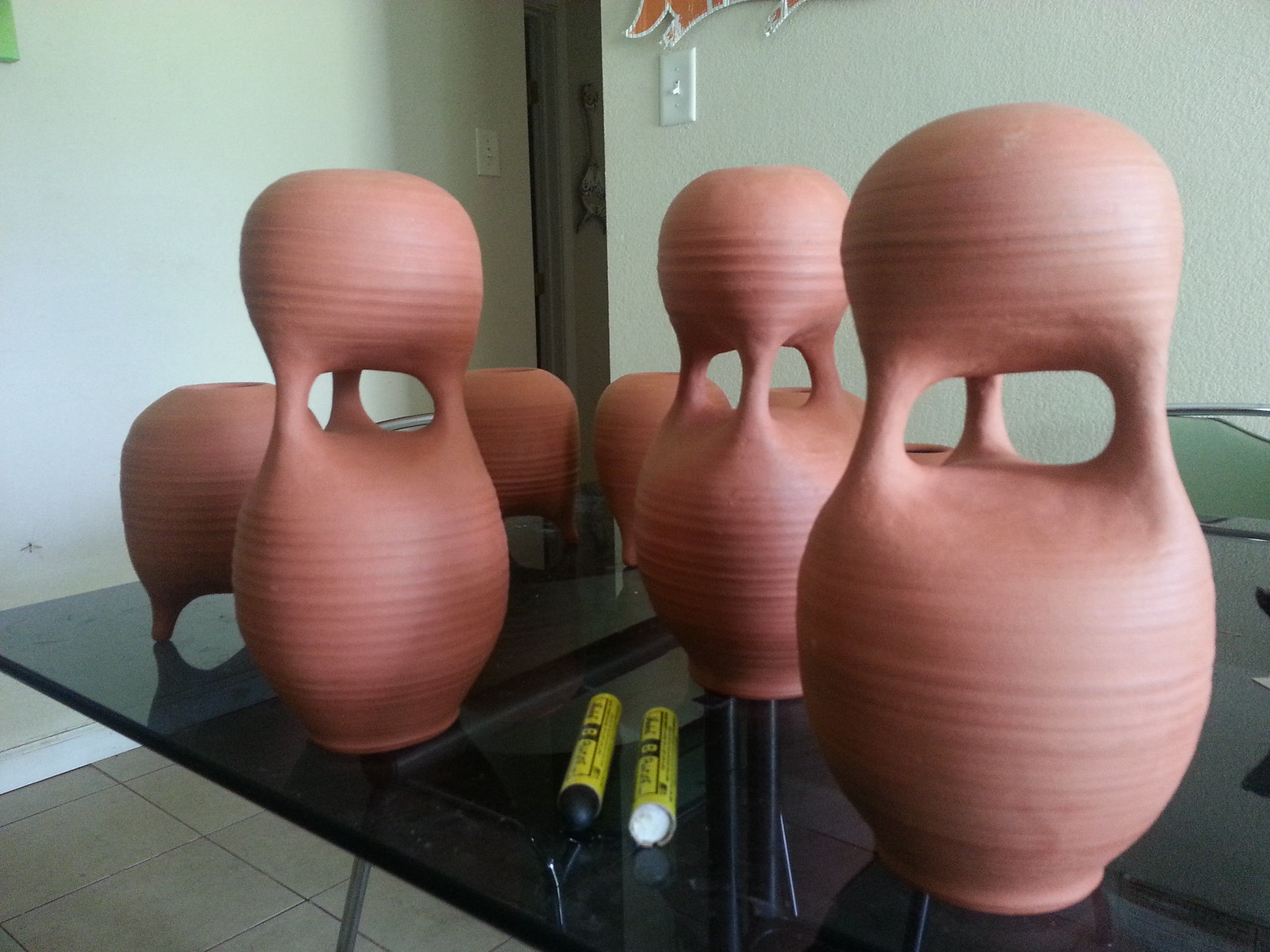The image depicts a room that appears to be an art class, characterized by its white walls and a mixture of light gray tones. Two light switches are visible on either side of the room, and a dark brown door is positioned in the corner. The focal point of the image is a large black glass table with metal legs, around which a couple of chairs are situated. Arranged both on the table and slightly behind it are various pottery sculptures made from a pinkish clay. These sculptures feature a unique design where three of them have a rounded base supported by three little legs and an oblong hole in the middle, giving them an appearance reminiscent of vases or abstract creatures with two eyes. Additionally, at the forefront, there are three larger sculptures with a similar design. Scattered on the table are two markers: one black and one white, as well as two yellow markers with black lids. The room has a cream-tiled floor, further enhancing the impression of a clean, creative space possibly used for crafting or teaching art. A whimsical touch is added by an object hanging on the wall resembling the legs of a small dog positioned just above one of the light switches.